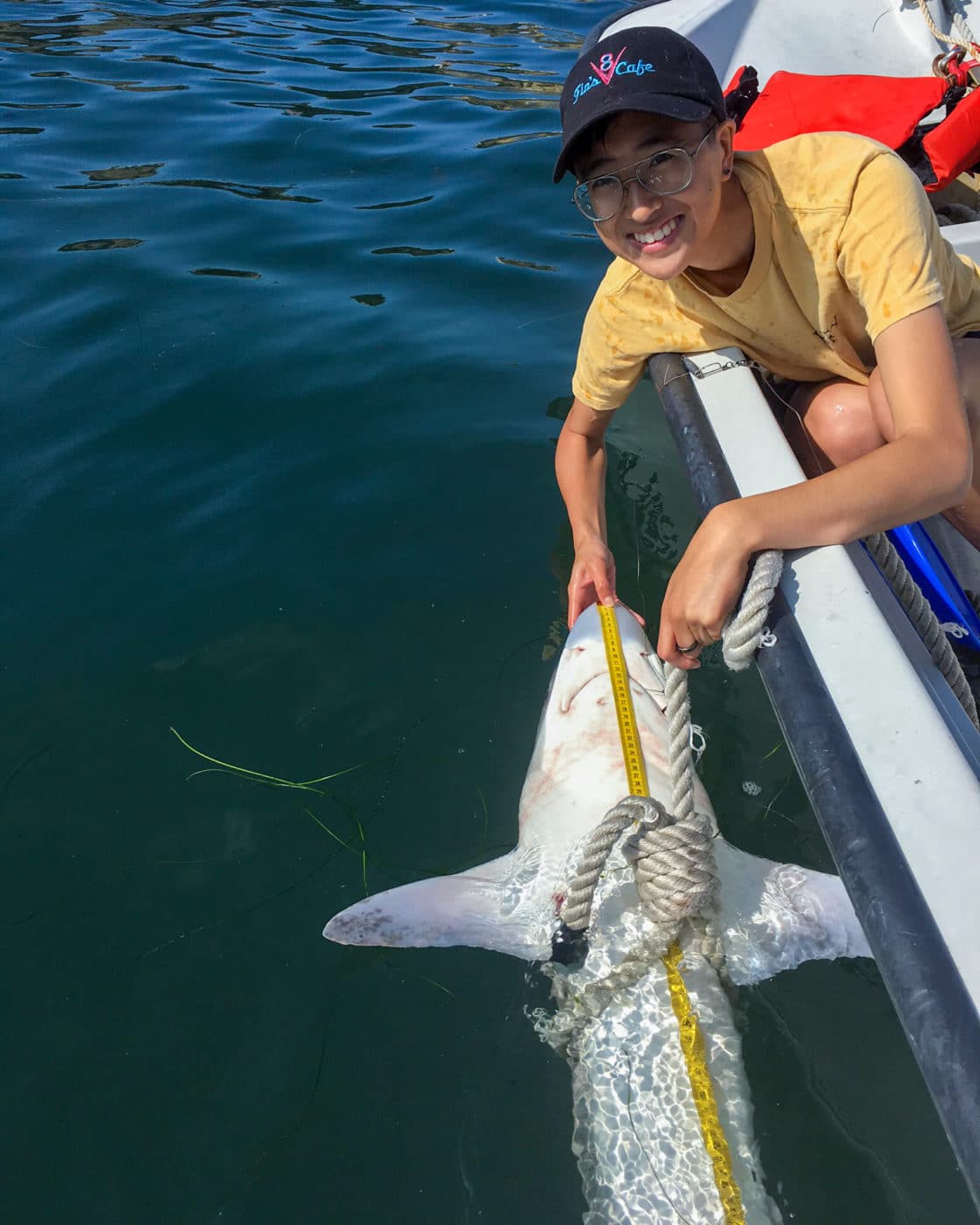In the image, a young, slender woman, possibly Asian and appearing to be a teenager, is seen on a small, white and black boat in murky waters. She is wearing glasses, a black baseball cap with some writing on it, and a yellow t-shirt. Her hair is either pulled back or very short and tucked under the hat. She is smiling brightly and appears to be having a good time. Crouched with her knees up to her chest, she leans over the edge of the boat, resting one forearm on the boat's ledge while holding a yellow measuring tape in her other hand. The tape measure is extended along the underside of a small shark, which is floating belly-up in the water. A rope, tied around the shark like a noose, secures it to the boat. It seems like she is measuring the length of the shark, which they likely caught while fishing. The scene captures a moment of excitement and curiosity as she engages in this fishing activity.